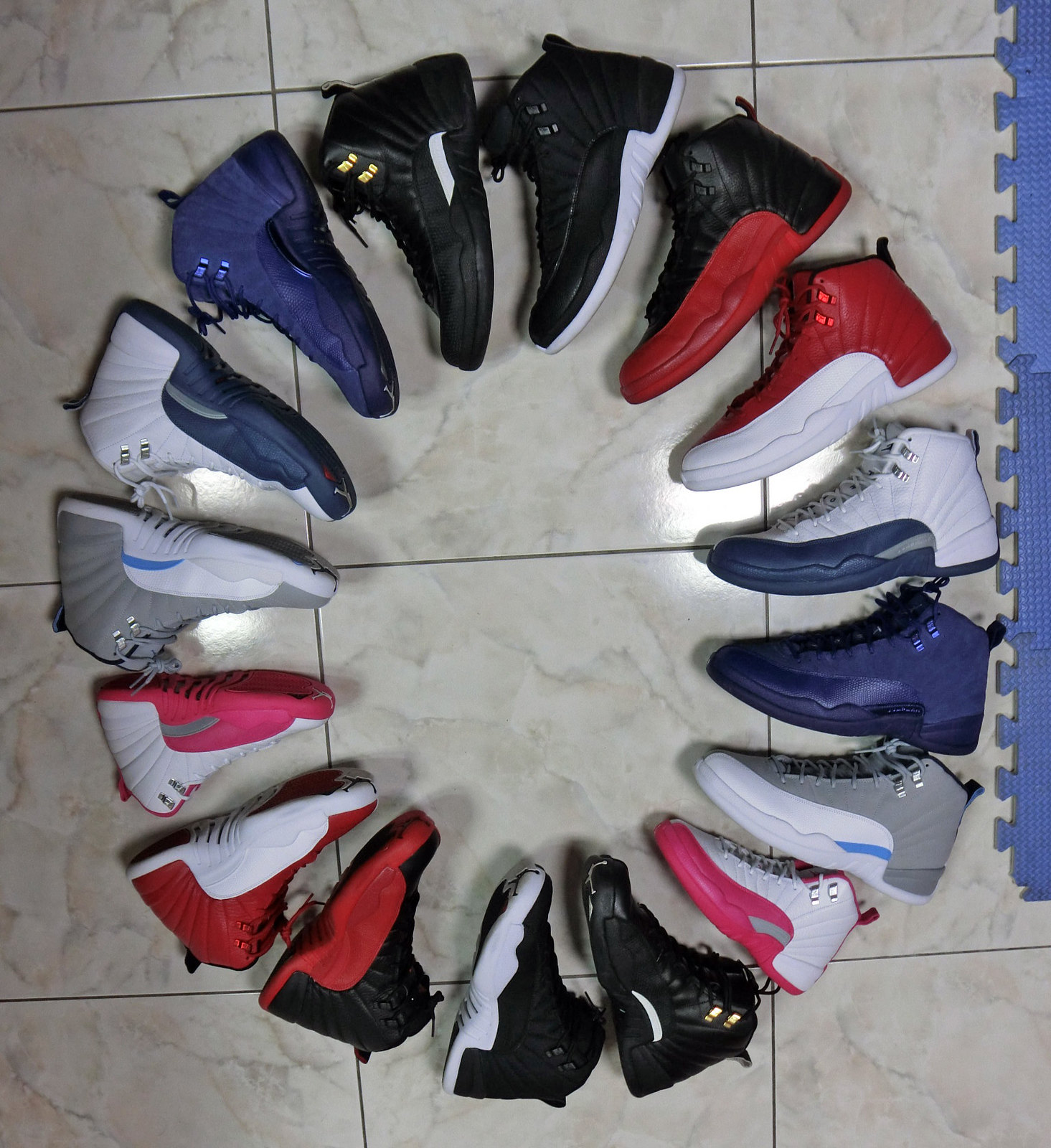The image showcases an overhead view of numerous pairs of tennis shoes meticulously arranged on a tiled floor. The floor tiles are predominantly white with light grey swirls, resembling a 12-by-12 inch pattern. Centered in the photo, the shoes form a precise circle, with each pair aligned directly opposite each other, their toes pointing toward one another at the circle's center. The shoes vary in color, including blue, black, gold, white, purple, gray, pink, and red. Noteworthy pairs include a black shoe with red accents, a purple shoe, a dark blue shoe, and several mixed-color pairs like white with purple, gray with white, and white with pink. To the right side of the circle of shoes, there is a foam exercise mat with interlocking edges, typically used in a home gym to protect the flooring from heavy weights. The shoes, resembling basketball styles that cover the ankles, total to eight pairs, making sixteen shoes arranged systematically.